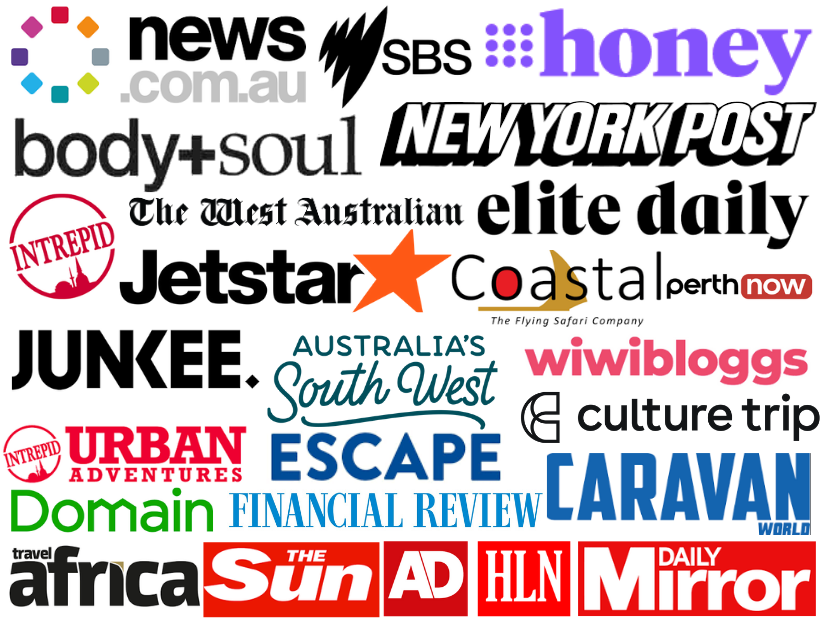A detailed and polished caption for the given image would be:

---

A collage screenshot featuring an array of multicolored icons representing famous websites, set against a white background. 

- Top Row:
  - The first icon on the left is from news.com.au, featuring a distinctive logo.
  - To its right is a gray icon for newsisblack.com.au.
  - A multicolored circular icon made of little squares is positioned to the left of these.
  - The SBS logo, a black thunderbolt, is situated to the right.
  - Further right, a blue dotted array spells out "honey."

- Second Row:
  - "Body and Soul" is depicted in a clean black font.
  - "New York Post" appears in a white font enclosed in black-bordered bubbles.

- Third Row:
  - "The West Australian" is shown in a classic newspaper-style font.
  - Next to it is the "Elite Daily" logo.

- Fourth Row:
  - A red circular logo featuring the word "Intrepid."
  - Below it, a simple icon representing church steeples.
  - The "Jetstar" logo in black font, with a red five-pointed star at the end of the word.

This organized arrangement highlights the diverse and recognizable logos of various well-known websites.